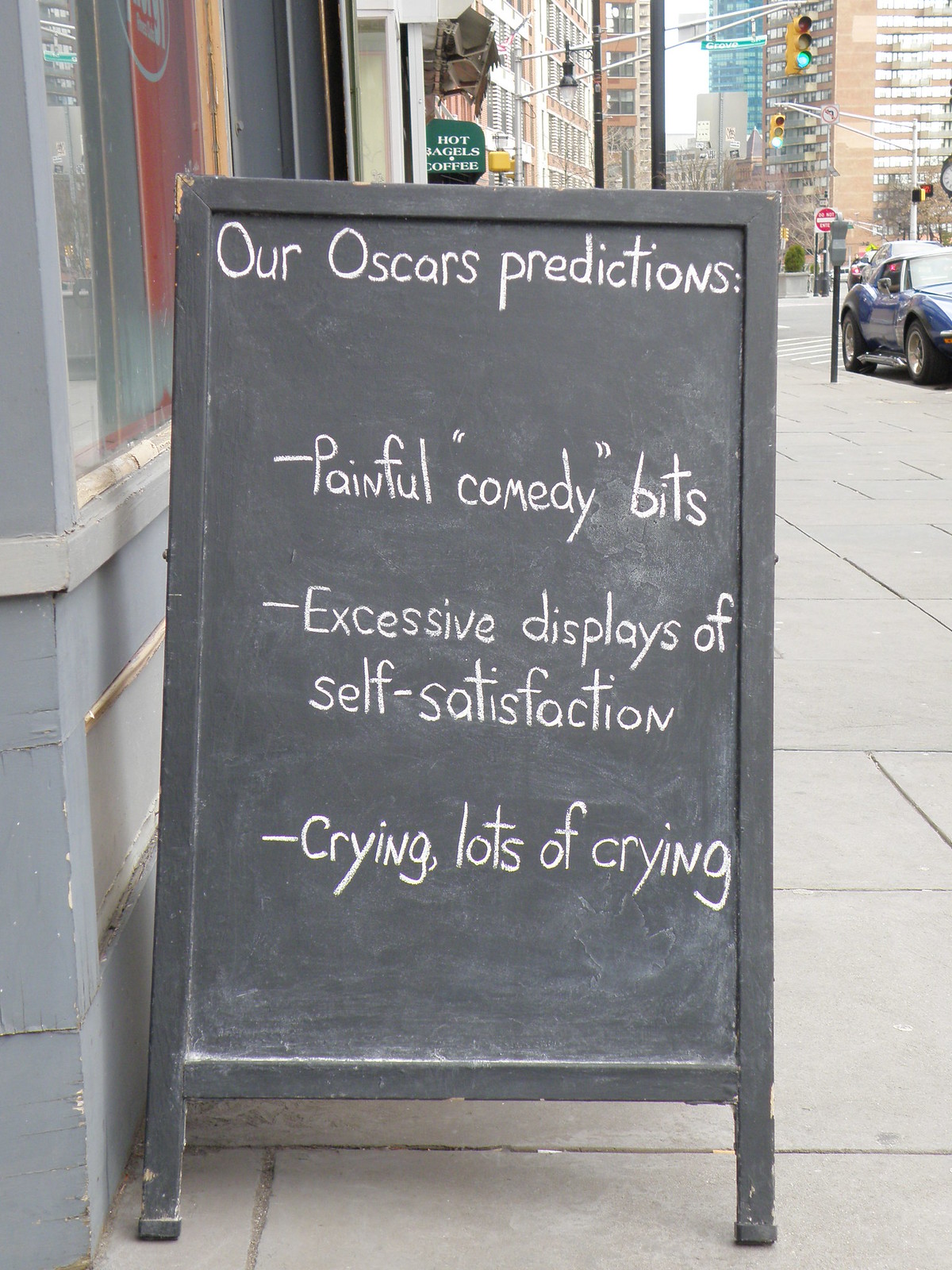The image depicts a humorous sandwich board sign standing on a wide city sidewalk in front of a business establishment. The black, four-legged sign has a chalkboard surface with handwritten text that reads, "Our Oscar Predictions: Painful Comedy Bits, Excessive Displays of Self-Satisfaction, Crying, Lots of Crying." The sign is placed under an awning that bears the name "Hot Bagels and Coffee" in white text on a green background. The bustling urban backdrop features tall buildings, a medium blue sports car parked by a parking meter, and various street signs including "Do Not Enter" and "No Left Turn." Two green traffic lights are also visible, adding to the city ambiance.